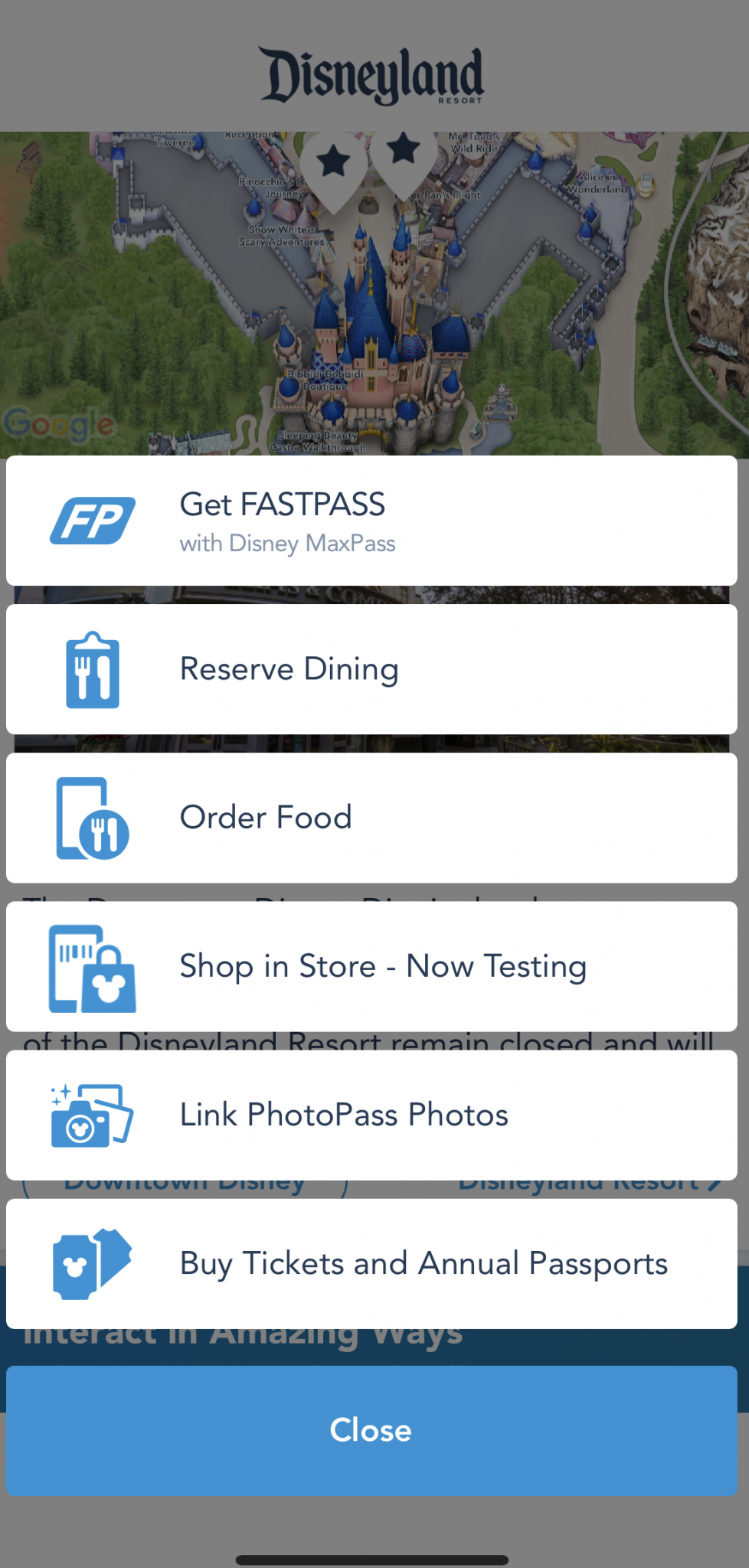This image captures the enchanting Disneyland castle standing majestically with a beautifully paved road meandering beside it, flanked by lush green trees. An array of icons and features overlays the picture, illustrating the park's convenient services. Prominently, a Fast Pass (FP) icon suggests using the Disney Max Pass for expedited access to attractions. Adjacent to it, a clipboard icon with a fork and knife encourages visitors to reserve dining options. A cell phone icon also bearing a fork and knife indicates the ability to order food directly from your phone. Highlighting the convenience of mobile shopping, another phone icon features a shopping bag with Mickey Mouse's head. For capturing memories, a camera icon with two blank pages suggests linking Photo Pass photos. Ticket purchasing is made easy, represented by two tickets, one adorned with Mickey's iconic head, symbolizing the option to buy both tickets and annual passports. The entire image is neatly framed, with "Close" prominently featured in white letters on a blue background, positioned above a black line at the bottom. The remainder of the descriptive writing is rendered in black, blending seamlessly with the overall design.